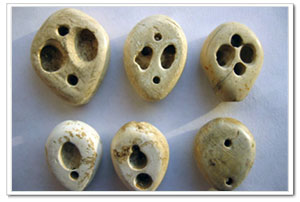The image features a set of six circular carvings made of stone, arranged in two rows against a gray background with a white rectangular border. The carvings, which appear polished and shiny, are mostly tan or off-white in color. Each stone carving is marked with holes of varying sizes and shapes. The top row consists of three carvings, each having two large oval holes in the center with smaller circular holes positioned at the top and bottom. In the bottom row, the first stone has a large singular hole towards the top and a smaller hole towards the bottom. The second stone features two equally-sized circular holes, while the third stone has two small holes. The carvings exhibit a consistent theme of perforations, although the positions and sizes of the holes vary, giving each piece a unique pattern.